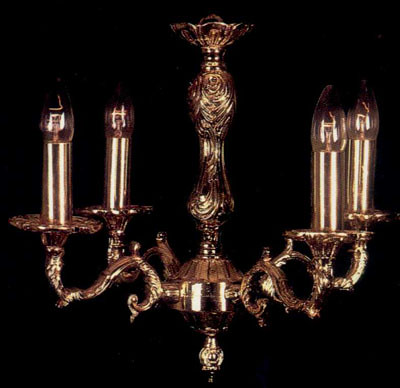This is a detailed color photograph of a chandelier-style light fixture set against a black background, designed to showcase the chandelier itself. The chandelier is made of a shiny metal that appears to have a brassy or potentially gold-toned finish, though the exact hue is difficult to determine due to the photograph's lighting. The central column of the chandelier supports four elegant arms that curve outward in an S-shape, reminiscent of tree branches. Each arm holds a flat base platform supporting a candle-shaped electric light bulb, creating a vintage aesthetic. The bulbs seem to be illuminated, casting a subtle glow that enhances the overall appearance. The chandelier is well-maintained, gleaming under the light, and the composition of the photograph makes it unclear if it is attached to a ceiling or if it is suspended in mid-air.